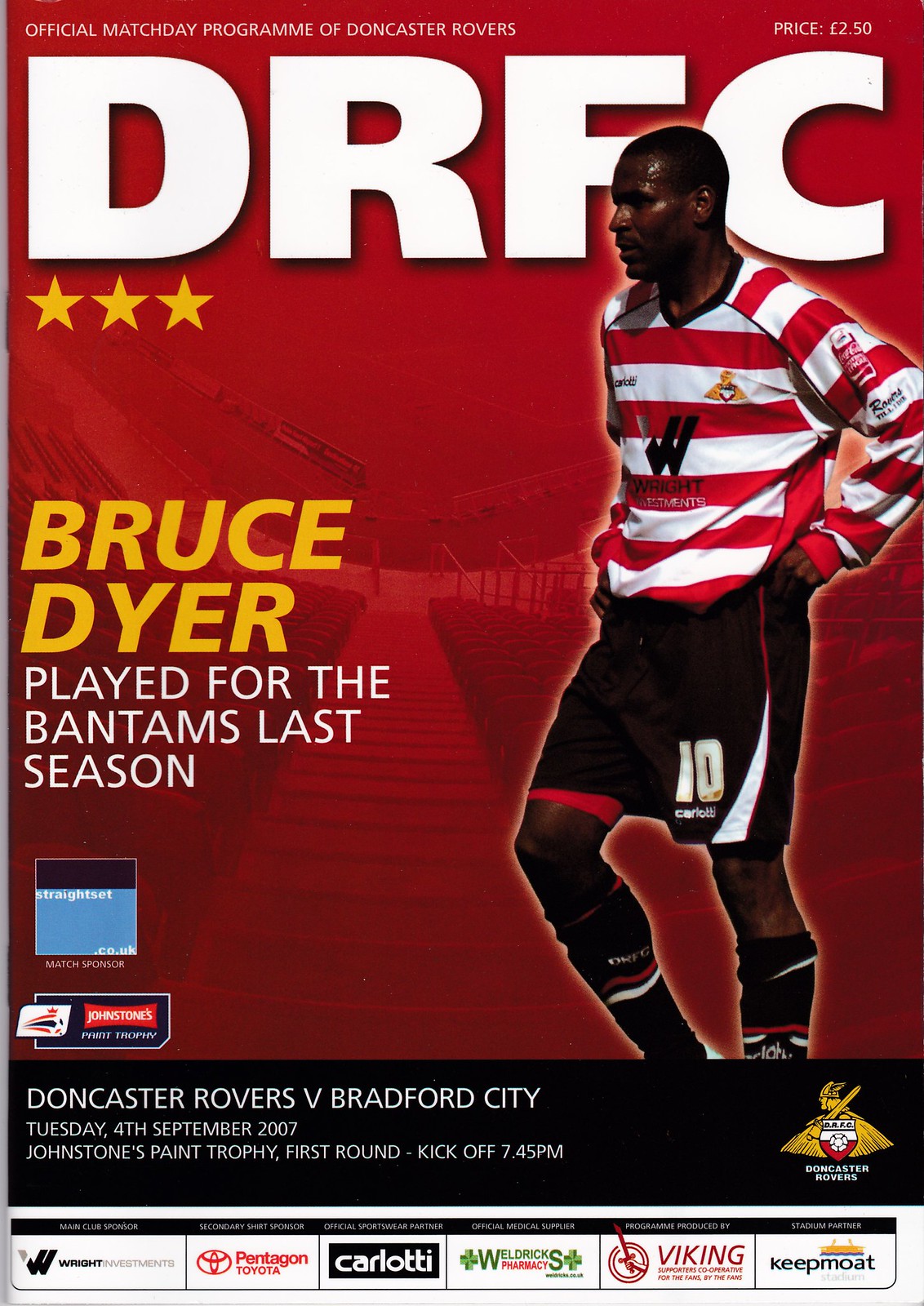The cover of this official Match Day program for the Doncaster Rovers is predominantly red, resembling a soccer stadium with a view from the top stair descending to the field. Central to the cover is an image of Bruce Dyer, a black man in a red and white striped long-sleeve jersey featuring a "W" on it, and black shorts marked with the number 10 on the left thigh. He appears to be in action, looking to his left, with a light glow surrounding him, emphasizing his dynamism. At the top, "DRFC" is prominently displayed in large white letters accompanied by three yellow stars under the "D," and just above, it reads "official match day program of Doncaster Rovers" in smaller white text. To the left of Dyer, large yellow text announces "Bruce Dyer," with a white caption below stating "played for the Bantams last season." The bottom of the cover features a black bar listing key match details in white text: "Doncaster Rovers v. Bradford City," the date "Tuesday 4th September 2007," the event "Johnstone's Paint Trophy first round," and the kickoff time "7:45 p.m." This bar also includes a gold insignia of a Viking holding a sword and shield with "Doncaster Rovers" beneath it, along with a row of sponsorship logos.